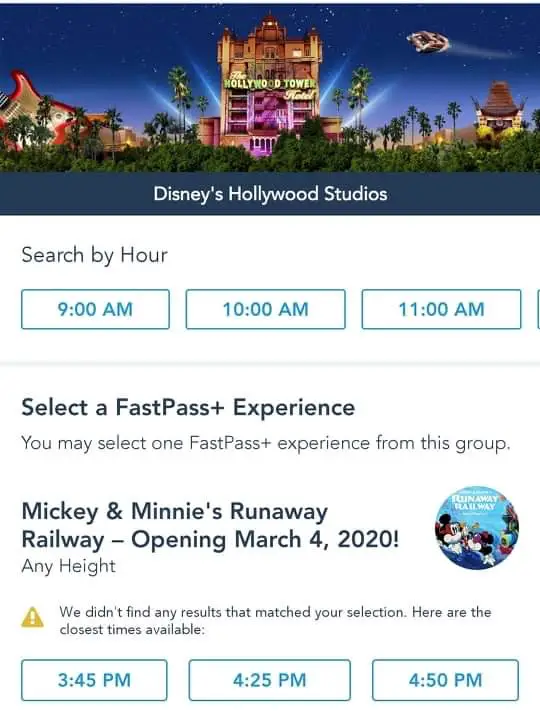The image is a vertically-oriented graphic, but its upper section features a horizontal rectangular picture of the iconic Hollywood Tower. The tower is depicted in a brownish hue, bearing the words "HOLLYWOOD TOWER" in prominent yellow, all-capital letters, with the word "hotel" placed underneath and slightly to the right. The tower's colors transition from an orangey-brown at the top to a pinkish tone towards the bottom. Surrounding the tower, luscious green palm trees stand against a starlit night sky.

Emerging from behind the hotel, radiant beams of light fan out diagonally towards the upper left and right corners of the image. Within the night sky, a mysterious flying vehicle heads toward the right. On the left edge, a partial red guitar is visible, cut off midway. To the right, a yellow figure wearing a cowboy hat is noticeable along the middle edge.

Beneath this scene, in black text, the words "Search by hour" appear above three turquoise-outlined rectangular boxes, offering selections of "9:00 a.m.," "10:00 a.m.," and "11:00 a.m." Following this, large bold black text reads "Select a FastPass+ Experience." It explains the selection options with the text "You may select one FastPass+ experience from this group."

Highlighted in bold black, it states "Mickey & Minnie's Runaway Railway - Opening March 4, 2020!" followed by "Any Height" in regular font. A yellow triangle with a white exclamation mark alerts: "We didn't find any results that matched your selection. Here are the closest times available." This message accompanies another set of turquoise-outlined boxes indicating available times of "3:45 p.m.," "4:25 p.m.," and "4:50 p.m." 

Adjacent to the "Mickey & Minnie's Runaway Railway" text, a turquoise circle contains an illustration of Mickey, with the text "Railway" visible in white font along the right edge.